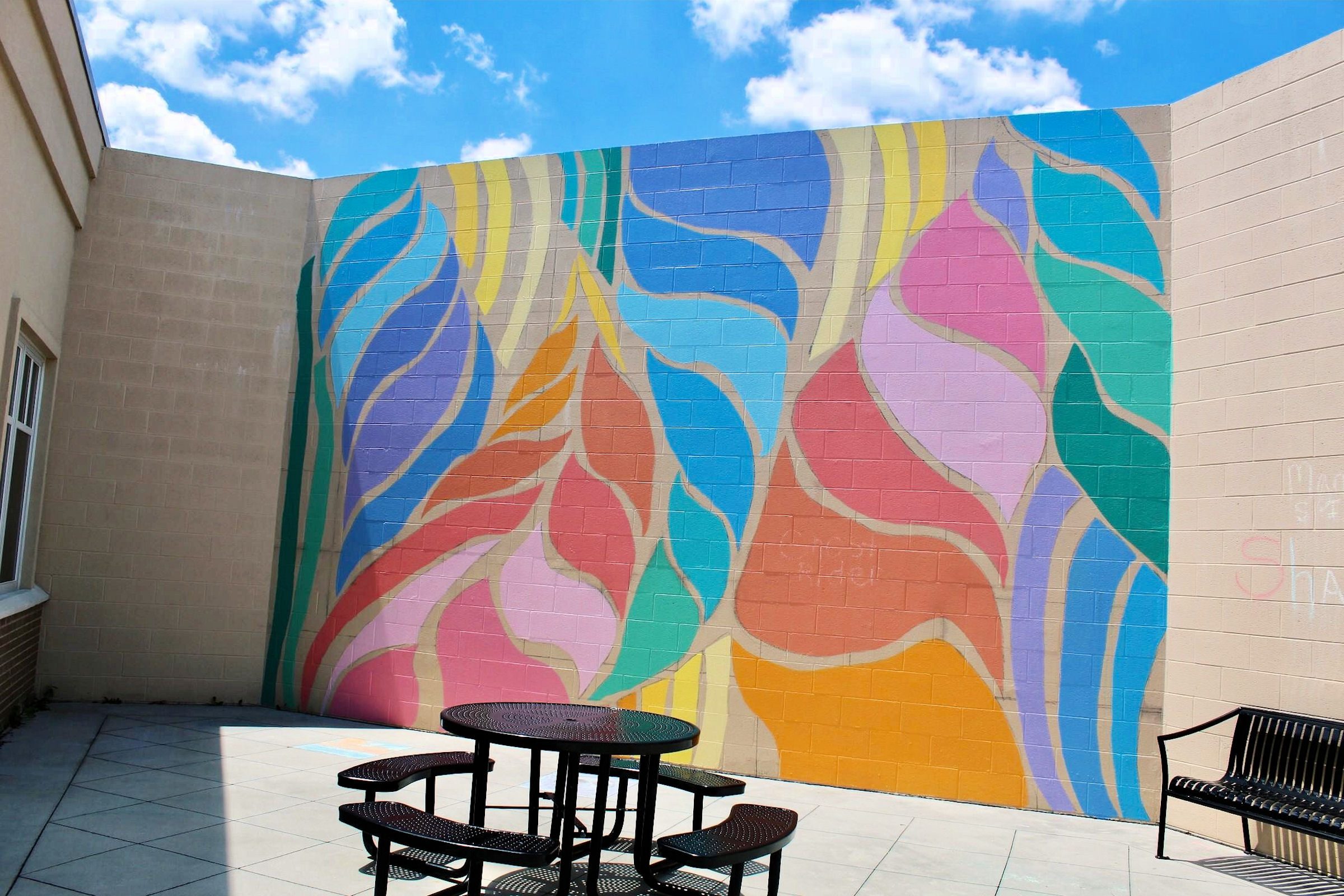This photograph captures a cozy courtyard space featuring a visually striking mural. The mural, which spans a large, light tan brick wall, is a vivid depiction of large, floppy leaves in an array of colors including varying shades of pink, orange, red, yellow, blue, purple, and green. These colorful leaves create a vibrant, botanical explosion that takes over the entire central wall. On either side of the mural, the walls are painted beige, completing the three-sided, trifold enclosure. 

In the foreground, set on cement pavers, stands a round black picnic table with four rounded, connected seats, offering a spot suitable for dining or relaxing. Additionally, to the right of the photograph, there is a black wrought iron bench positioned against the mural-covered wall. The overall setting is brightened by a sunny sky with puffy white clouds that adorn the backdrop, adding to the cheerful atmosphere of this inviting courtyard.